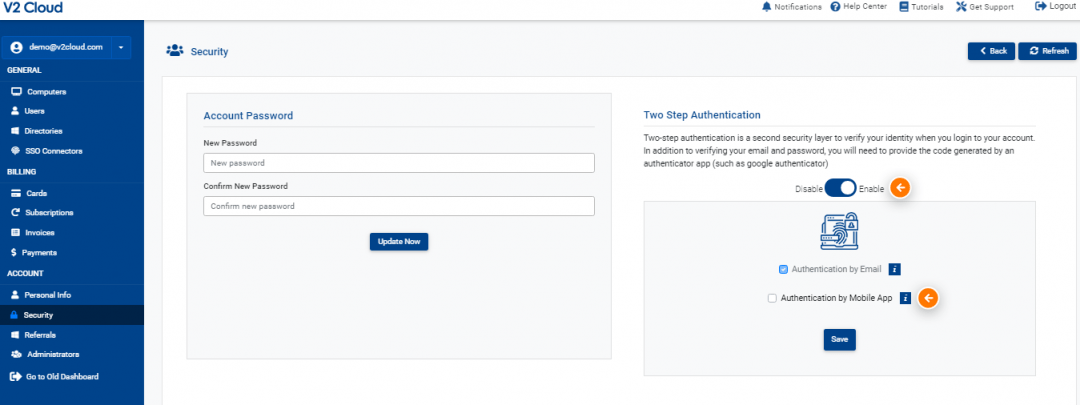The web page titled "V2 Cloud" features a top navigation bar with a white background, where "V2 Cloud" is prominently displayed in a blue font on the top left corner. Adjacent to this header, a vertical column spans the page's left side, adopting the same shade of blue as the "V2 Cloud" text. This blue column serves as a navigation menu, listing various site links and directories in a contrasting white font.

The main section of the page features a gray background with a slightly pinkish hue. At the top of this section, the word "Security" appears in a blue font against a gray background strip. To the right of this word are two buttons: a blue back button with white text, and a refresh button with white text on a blue backdrop.

Beneath this, a login form is presented, prompting users to enter and confirm their new passwords in white input boxes. Instructions and form labels, such as "Account Password," are displayed in a blue font. A prominent "Update Now" button is situated at the bottom of the form, distinguished by a blue rectangle and white text.

To the right of the form, directions for two-step authentication are provided in a blue font, accompanied by options to enable or disable this security feature, with choices highlighted in blue and white.